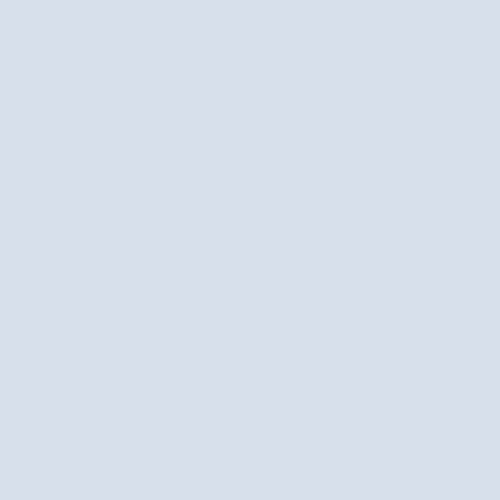A solid gray-blue square occupies the entire frame. There are no additional visual elements, indicating either a loading error, a server-side failure, or a deliberate test of attention. The square is uniform in color without any discernible patterns or textures, leaving the viewer without further context or interactive options.